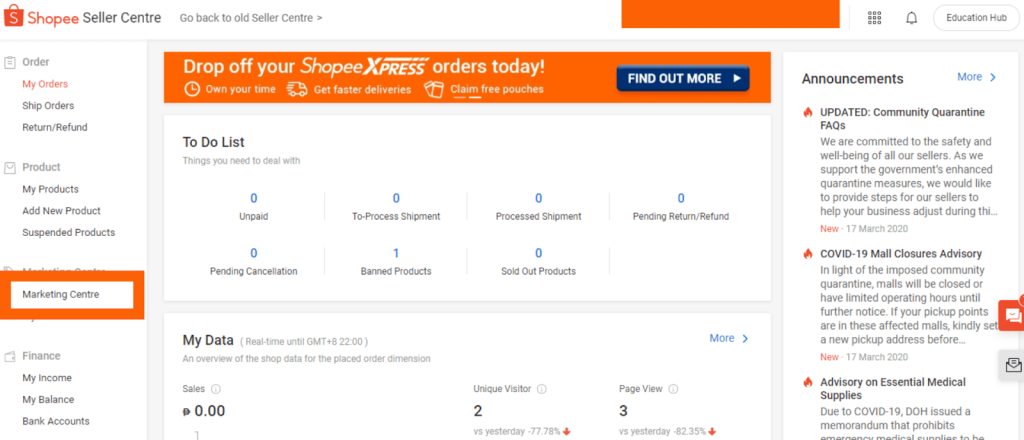This image depicts a webpage from the Shopee Seller Center. In the upper left-hand corner, the Shopee logo, featuring an orange shopping bag with a white "S" and the word "Shopee" in orange, is prominently displayed. The header also includes the text "Seller Center" written in black and an option to "Go Back to Old Seller Center" with an accompanying arrow.

On the right side, there's a long orange navigation box. Beneath the central section of the webpage, a banner invites users to "Drop off your Shopee Express orders today," with a blue button labeled "Find Out More" and an arrow indicating additional information.

Further down, a to-do list is visible, highlighting various tasks such as managing sold-out products and shipments. Each task is accompanied by numerical indicators, written in blue. Another section labeled "My Data" provides access to user statistics, with a "More" button available for additional details.

On the left side of the page, a vertical navigation column lists sections like "Order," "Product," each expanded to show subcategories. The "Marketing Center" is particularly highlighted with a thick orange outline. Additionally, "Finance" is broken down into "My Income," "My Balance," and "Bank Accounts."

On the right side of the page, the "Announcements" section is prominently featured, with a "More" link in blue next to the title. This section includes an update about COVID-19 and an advisory on essential medical supplies.

Overall, this detailed webpage layout provides a comprehensive interface for sellers managing their Shopee accounts.